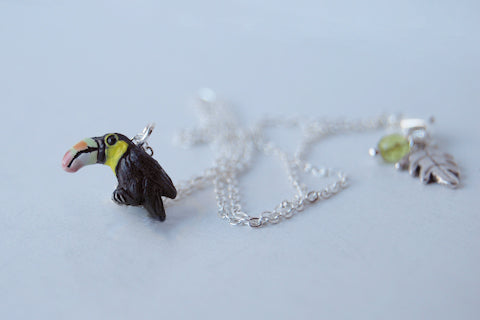This photograph showcases a close-up view of a silver charm bracelet placed on a light blue surface that fills the background. The bracelet's chain is positioned in a somewhat disorderly manner, with it blurred in parts, particularly the back half. On one end of the chain, there is a detailed pendant of a black toucan bird facing to the left. The bird features a light white beak adorned with a peach-colored stripe, a black eye encircled by a subtle yellow ring, and yellow patches on its neck and arm. The beak displays a gray color with a distinguishing black stripe down the center separating the top from the bottom, and a hint of a very pale pastel red along the top. The other end of the chain is connected to a leaf-shaped charm, which is silver with jagged edges, detailed lines, and includes a translucent bead hanging off the left side of the charm. The leaf appears to be tinted slightly with pink and white hues, contributing to the intricate design of the bracelet.